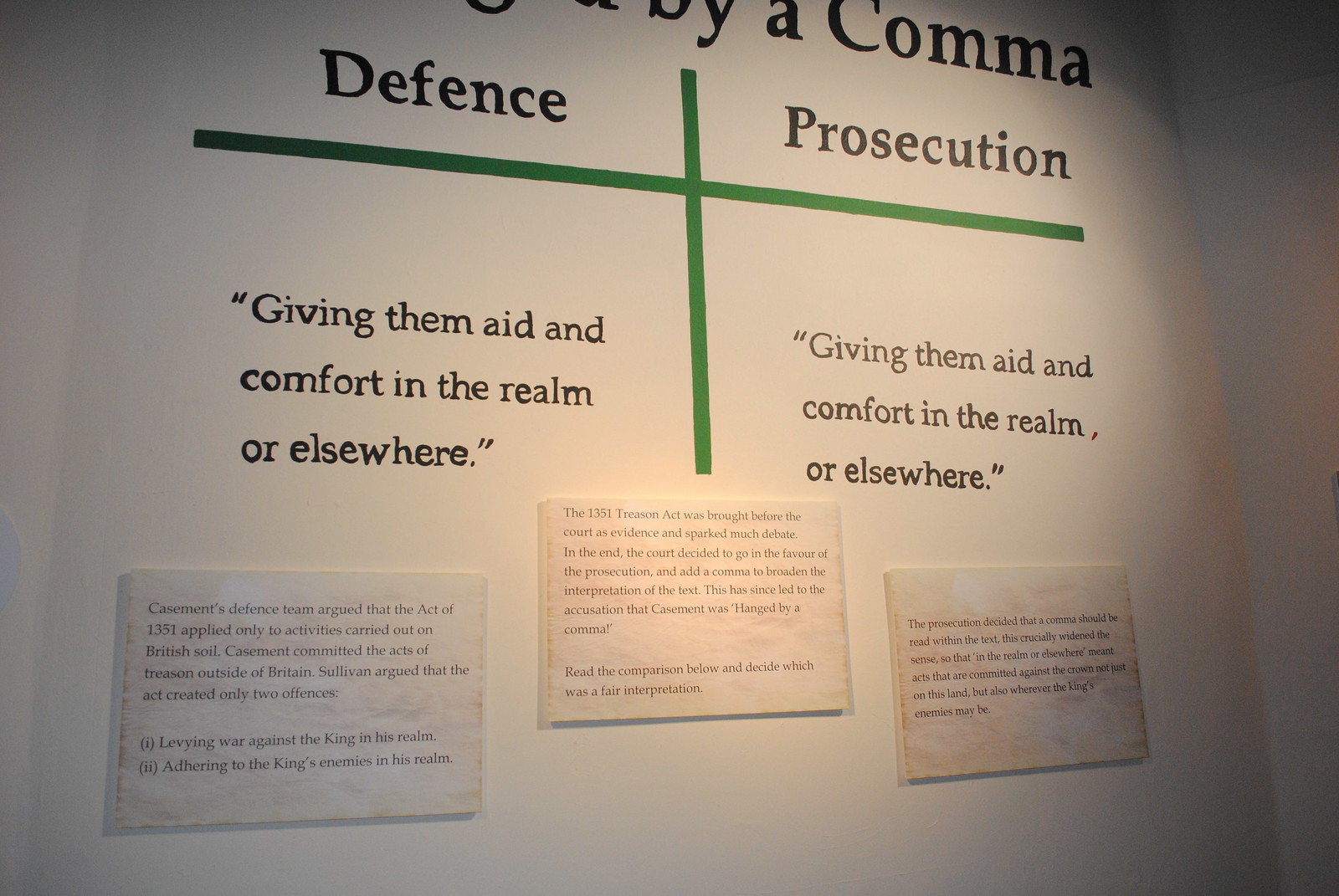The photograph depicts a white wall used as a detailed visual aid to compare legal interpretations. At the top of the wall, the words "Defense" and "Prosecution" are prominently displayed, separated by a green vertical line and underscored by red and green horizontal lines to form a tabular column. Below the word "Defense," the text reads "giving them aid and comfort in the realm or elsewhere," mirrored exactly under "Prosecution."

Fixed to the wall are three white papers featuring black printed text. The first block of text discusses how Casement's defense team argued that the 1351 Treason Act applied only to activities on British soil, insisting that Casement's acts of treason were committed outside of Britain. A specific mention is made of Sullivan, who argued that the act created only two offenses: levying war in the king's realm and adhering to the king's enemies within the realm.

The second block of text elaborates that the 1351 Treason Act was debated in court, with the final decision favoring the prosecution by adding a comma to the text. This addition broadened the act's interpretation, suggesting that treasonous acts committed against the crown were not confined to British soil but could occur "in the realm or elsewhere." Consequently, this change led to the historical accusation that Casement was "hanged by a comma." Visitors are invited to review the comparison and decide which interpretation they find fairer.

The setup, with its green crosses and meticulous text blocks, resembles a school project or a lawyer's methodical preparation for a case, providing an informative and engaging overview of a legal historical case.